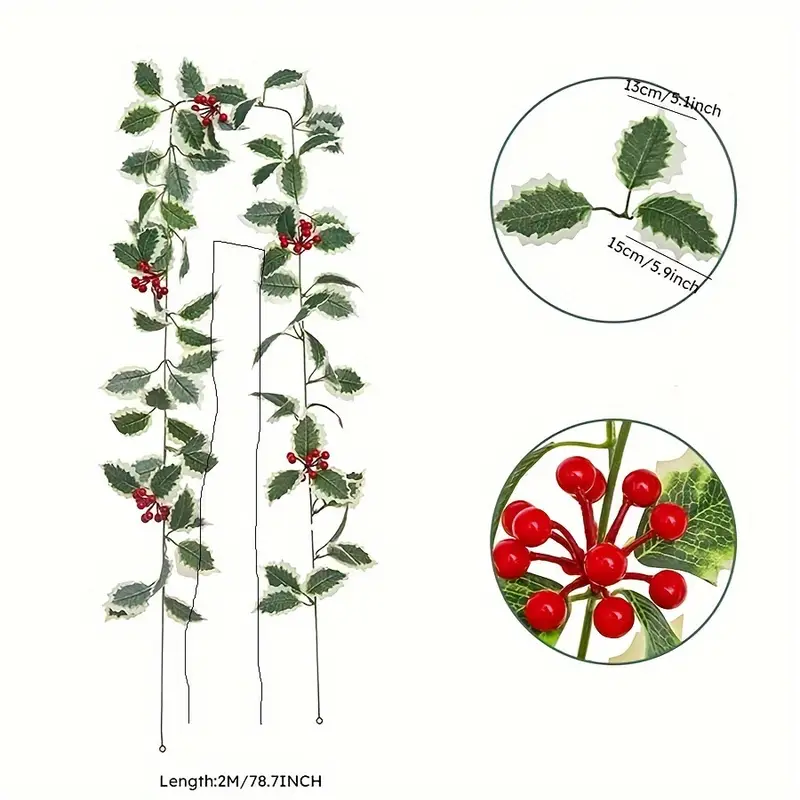The image showcases a detailed product display of an artificial cranberry vine. The left side features a vine with two large trunks adorned with long white rods, from which green leaves and clusters of red, glistening cranberries hang. These berry clusters are dispersed across the upper, middle, and lower segments of the vine, held together by red stems. The vine measures 2 meters (78.7 inches) in length. On the upper right, a close-up shows the intricate detail of the leaves, which are described as being 13 centimeters (5.1 inches) wide and 15 centimeters (5.9 inches) long, illustrated within a black circle. The bottom right part of the image provides a detailed view of the berries, demonstrating how they sprout from the central stems in circular formations. The background of the entire image is white, ensuring that the features of the vine, leaves, and berries are clearly visible.